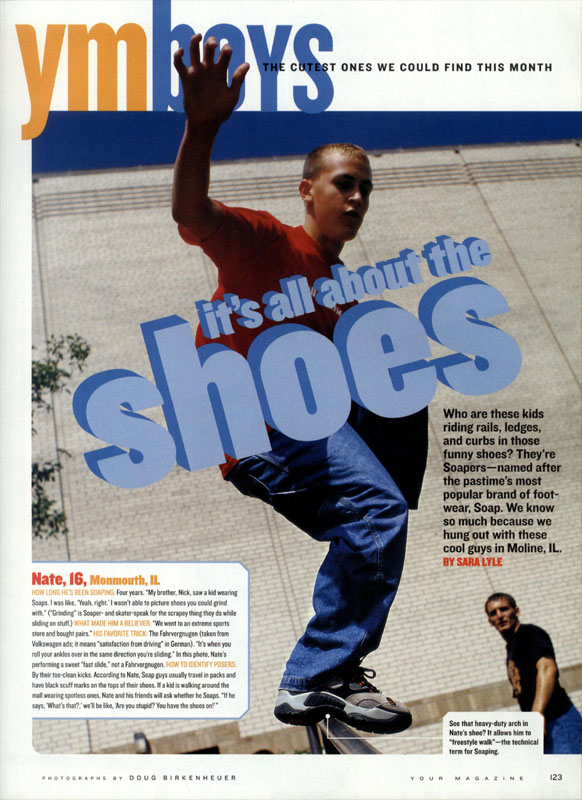This image is a rectangular magazine page taller than it is wide, appearing as if it has been ripped out. At the top of the page, a white header displays "YM" in yellow print and "boys" in blue print, combining to read "YM boys." Just beneath this, in small black print, it states, "the cutest ones we could find this month." The majority of the image is taken up by a photograph of a skateboarder, who is standing on a rail often found near staircases, with just his shoes visible. His face is obscured in shadow, but he appears to be a Caucasian teenager with short blonde or brown hair, dressed in a red short-sleeved t-shirt and baggy blue jeans. 

Dominating the center of the photograph, blue bold text proclaims, "it's all about the shoes." To the right of this, in black print, the caption reads, "Who are these kids riding rails, ledges, and curbs in those funny shoes? They're soapers, named after the pastime's most popular brand of footwear, Soap. We know so much because we hung out with these cool guys in Moline, Illinois." This text is attributed at the bottom to Sarah Lyle in red print.

In the lower left, a white bubble contains red print, identifying a boy named Nate, aged 16, from Monmouth, Illinois, followed by a brief paragraph about him. The footer of the page credits the photographs to Doug Birkenhauer and includes a faint mention of "your magazine" and the page numbers 1, 2, 3 on the bottom right.